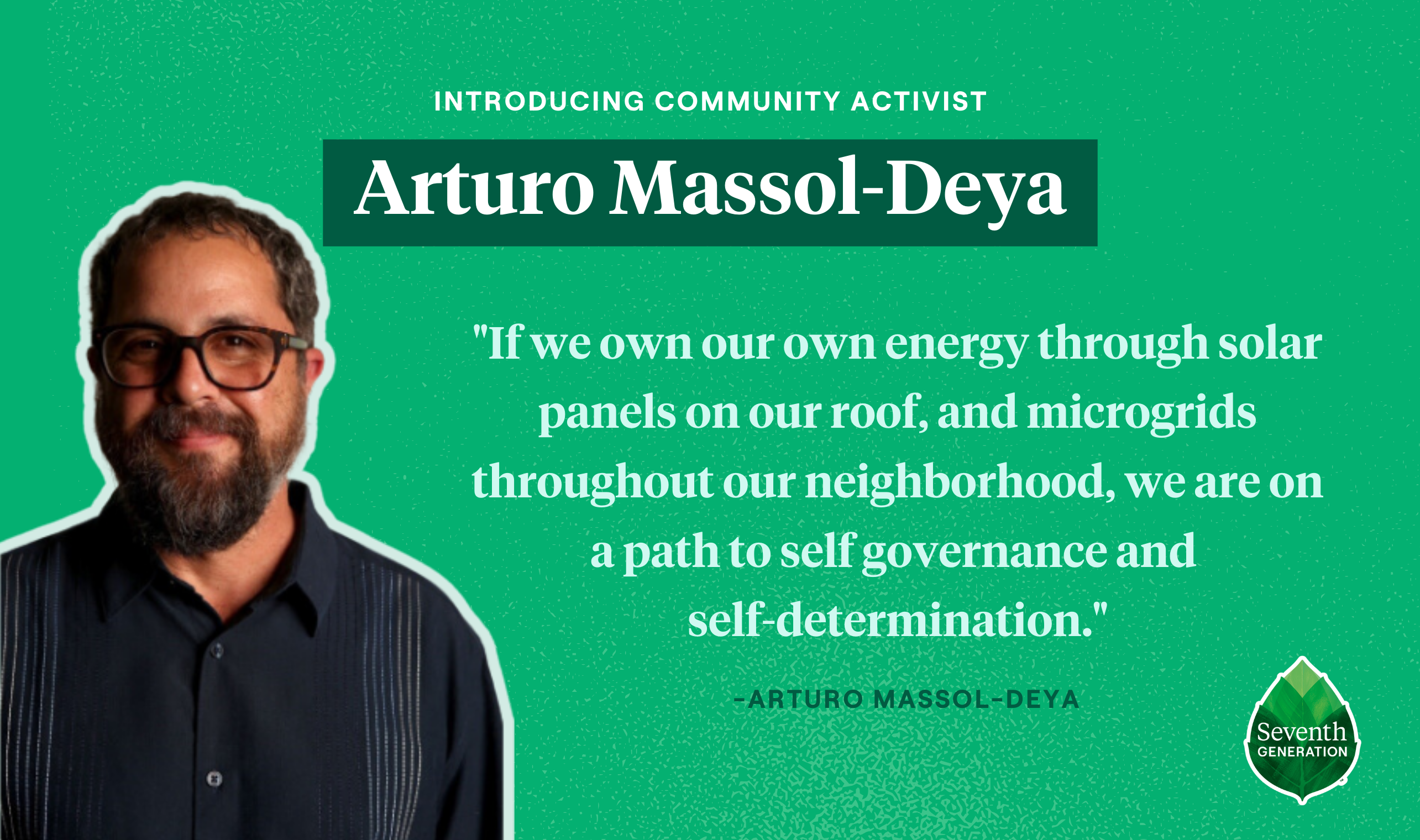The image features a banner with a mint green background and a portrait of a man on the left side. The man, identified as Arturo Masol-Dea, is depicted with graying black hair, a graying brown goatee, black-rimmed glasses, and a blue button-down shirt with white vertical pinstripes on each shoulder. He is smiling and looking directly at the camera. Above his head, there is bold white text saying, "Introducing community activist Arturo Masol-Dea." Beneath this, a quote attributed to Arturo reads, "If we own our own energy through solar panels on our roof and microgrids throughout our neighborhood, we are on a path to self-governance and self-determination." At the bottom right corner of the banner, there is a logo of a green leaf with the text "Seventh Generation" in white. The overall theme of the banner centers on community empowerment and sustainable energy initiatives.